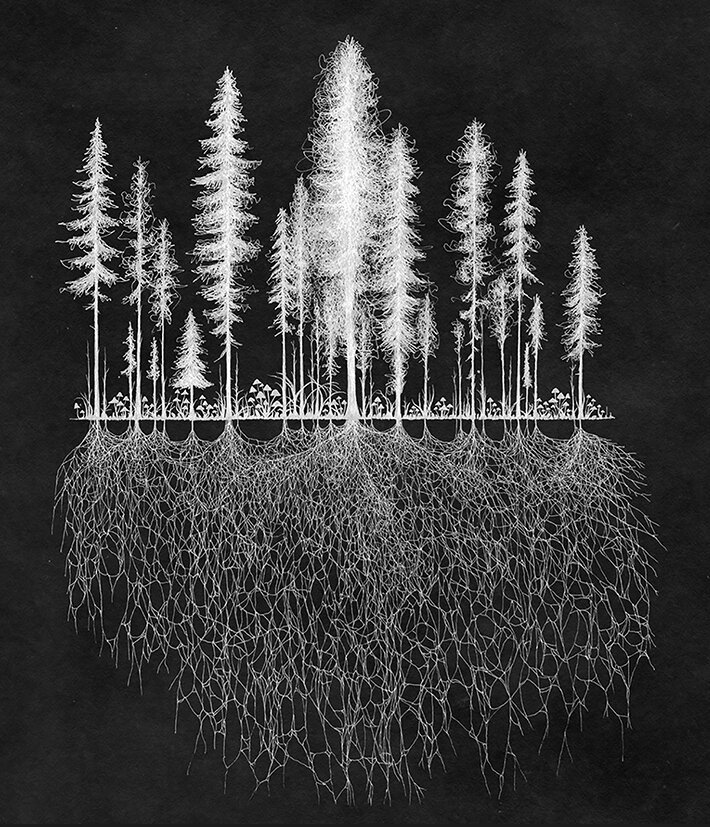This is a black-and-white artwork depicting a forest scene set against a large black background. The image features a line of approximately 20 white pine trees, arranged in a symmetrical pattern where the smallest trees stand on the far left and right edges, gradually increasing in height towards the center. The tallest tree is centrally placed, with smaller trees and even some mushrooms scattered along the forest floor between them. The forest floor itself houses ferns and other vegetation, all rendered in white. Below the ground, the illustration reveals an extensive and intricate root system that mirrors the trees above. These roots intertwine and extend deep into the soil, resembling a spiderweb, and cover about half of the picture, emphasizing the connectedness and complexity of the natural world above and below the ground.